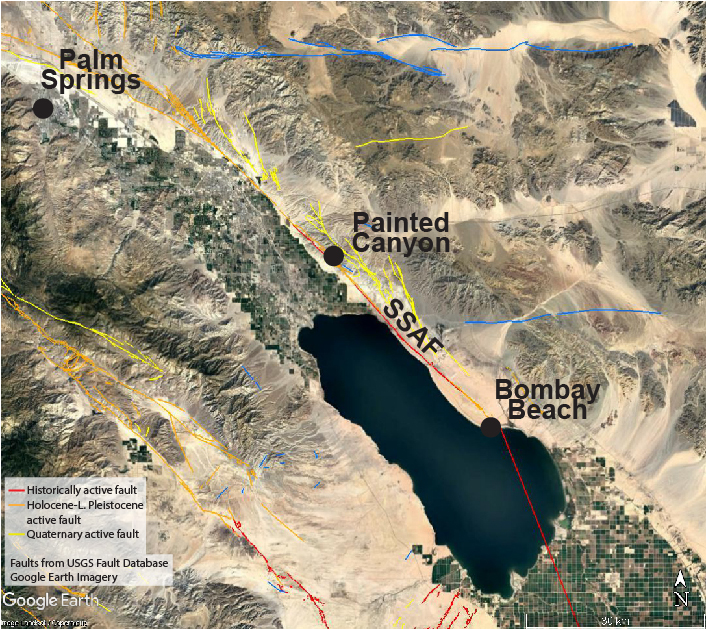This is a detailed Google Earth satellite image featuring a desolate desert landscape dominated by a black-colored body of water situated in the lower right. Surrounding the water on the left are extensive mountainous terrains, identifiable by their textured gray elevations and a stark lack of greenery. The region around the water has some green patches, specifically on the lower right and upper left sides. To the upper right of the water lies flatter, sandy terrain with some hills. Black text labels several key locations, including "Bombay Beach," positioned right next to the water, "Painted Canyon," "Palm Springs," and "SSAF," which is indicated with a red line. An index found on the lower left of the image, labeled "Google Earth," lists various fault lines—highlighted in multiple colors (yellow, red, and blue)—and terms such as "historically active fault," "Holocene," "L-Pleistocene," and "quaternary active fault" from the USGS fault database. This high-altitude aerial view captures a barren, brown-hued environment marked by rugged mountain ridges devoid of snow and dense vegetation.